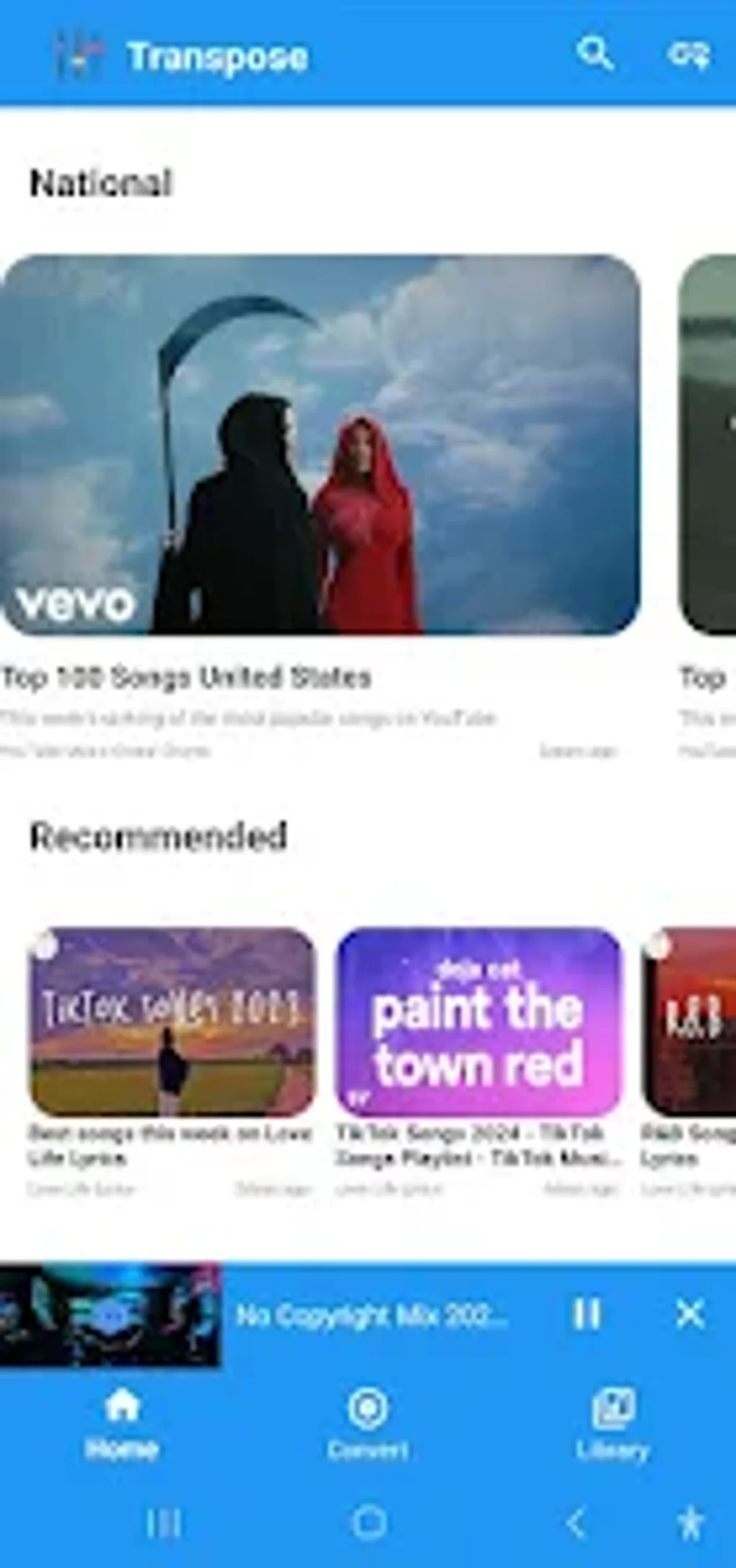This is a detailed caption for the provided image:

---

A screenshot from an unspecified app or webpage features a blue border at the top with the word "Transpose" inscribed in white text next to a white magnifying glass icon. Below this header, the word “National” is visible. The main content of the screenshot showcases an image of the Grim Reaper holding a scythe, standing beside a woman in a red dress. They are set against a backdrop of a blue sky with scattered clouds. In the bottom left corner of the image, the text "VEVO" is displayed in white letters. Beneath it, the phrase "Top 100 Songs United States" is legible, followed by some blurry, unreadable writing. 

Further down the screen, the word “Recommended” appears. There are blurred texts, including a mention of "TikTok". Another portion of the text reads "Paint the Town Red" but is followed by more unreadable writing. The bottom section of the screenshot features a blue rectangle containing the phrase "No Copyright Mix", along with a row of icons: a pause icon, an X icon, a home icon, a connection icon, and a library icon. 

At the very bottom of the screen, three thin vertical lines, a white circle, a left-pointing white arrow, and a white star are aligned. The overall image has a portrait orientation, being taller than it is wide.

---